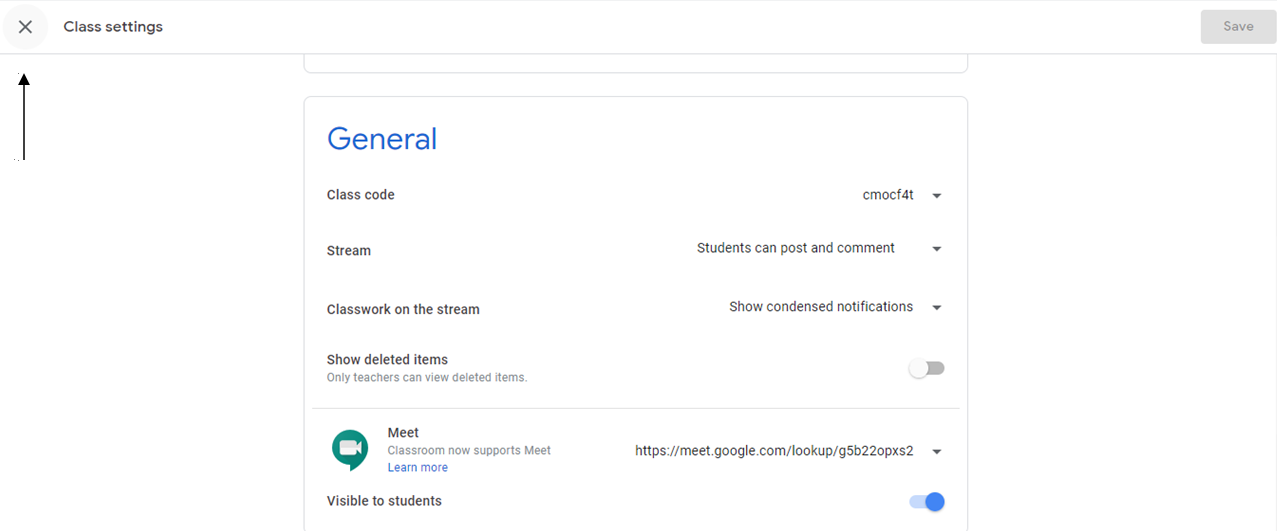The image depicts a settings window for an application, likely related to classroom management. The entire interface is set against a white background. At the top left corner, the header reads "Class Settings," and in the top right corner, there is a grey button labeled "Save," which appears to be inactive.

In the center of the page, there is a grey-outlined box featuring prominently the word "General" in blue. Within this section, users can configure four different functions:

1. **Class Code:** A drop-down menu that currently displays the code "C-M-O-C-F-E-I."
2. **Stream:** Another drop-down menu with the selected option "Students can post and comment."
3. **Class Work on the Stream:** A drop-down menu showing "Show condensed notifications."
4. **Show Deleted Items:** This option is controlled by a slider, which is currently set to deactivate, preventing deleted items from being displayed.

Below these settings, a dividing line separates the next segment, which includes a function labeled "Meet for Classroom." This feature seems to support video functionality, as indicated by its name. The "Support Meet" option is currently active.